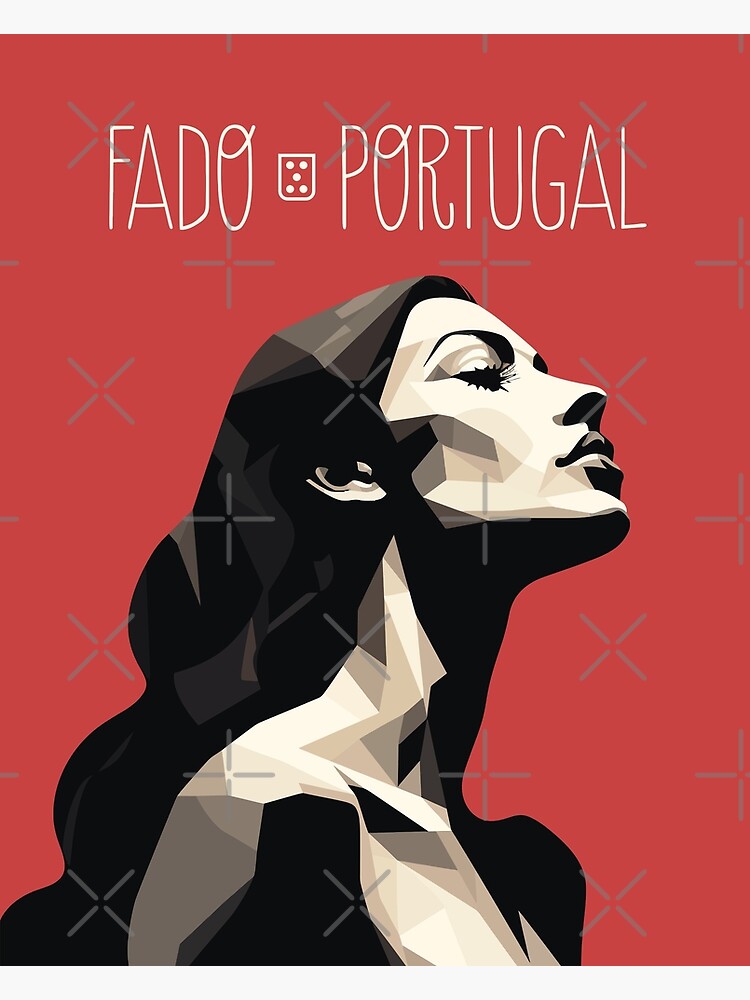This vertically aligned rectangular poster showcases a striking computer-generated design with a muted, brick-red background. At the top of the poster, thin, condensed white text reads "FADO, PORTUGAL," separated by a small crest resembling the front side of a dice with five dots. The majority of the poster is dominated by a geometric, black-and-white illustration of a woman, depicted from the shoulders up. She faces the top right with her chin tilted upward and her eyes closed, highlighting her long black hair and prominent eyelashes. The woman's body, formed with a collection of geometric shapes and silhouettes, gives a modern, artistic feel to the image. Subtle gray lines crisscross the background, forming patterns of X's and plus signs, possibly to indicate rights protection for the artwork.